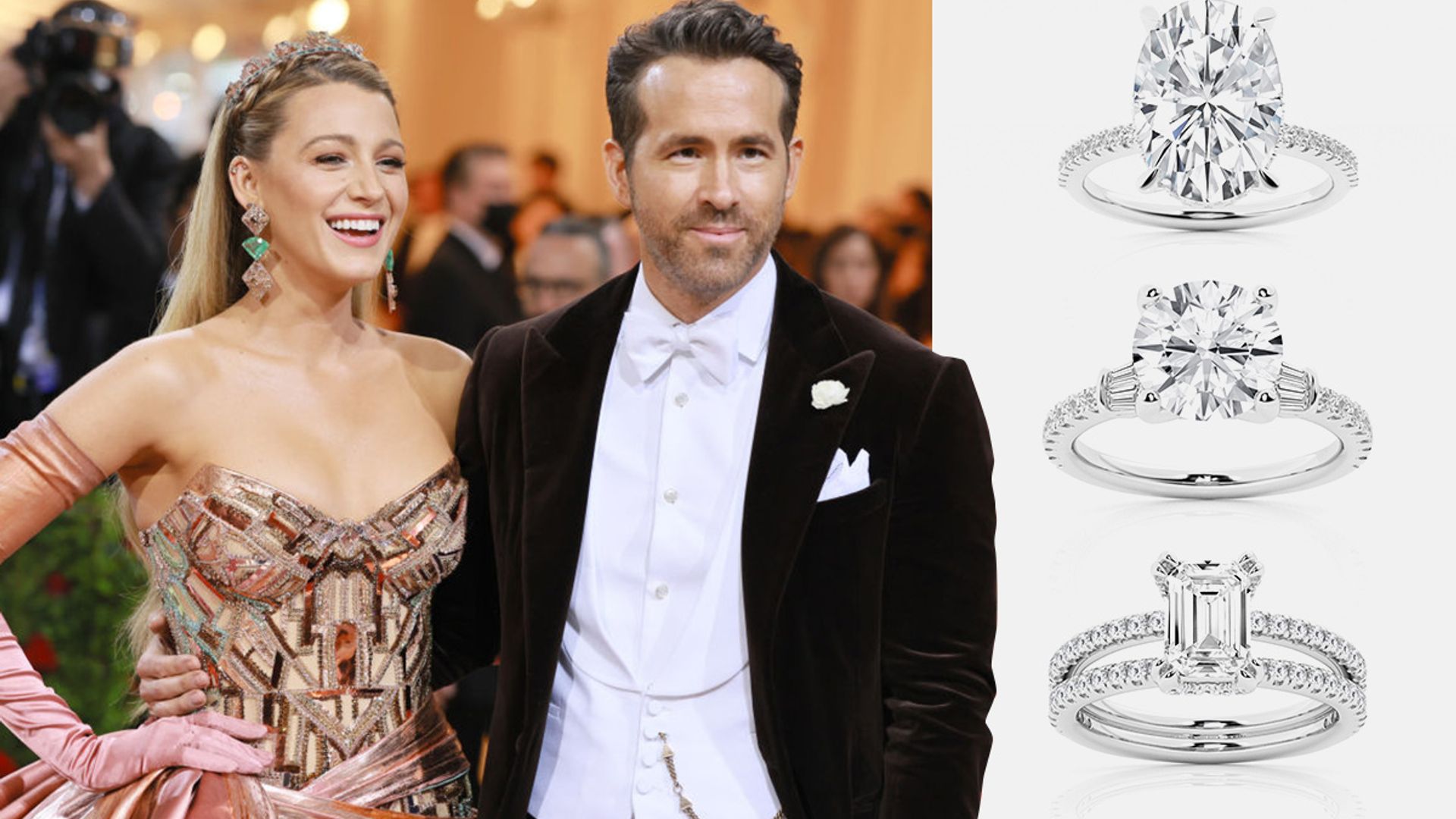This is a composite image featuring a photograph on the left side, which takes up about 66% of the picture, and a series of three diamond ring images on the right. The photograph shows famous actor Ryan Reynolds and his wife, actress Blake Lively, at a glamorous event, possibly the Met Gala or an award show. Both are captured from the waist up with a slightly blurred background filled with seated attendees and one person taking a photo behind them. Blake Lively, positioned on the left, is adorned with a tiara, dangling sparkling earrings, and a strapless dress that features a geometric pattern with shades of gold, beige, brown, and pink. She completes her elegant look with light pink gloves. Ryan Reynolds stands to her right, wearing a sophisticated black velvet tuxedo, along with a white shirt, white bow tie, white pocket square, and a white flower pinned to his lapel.

On the right side of the image, three diamond rings are showcased. The top ring features the largest diamond, which is oval-shaped. The middle ring has a medium-sized circular diamond, and the bottom ring displays a smaller rectangular diamond set vertically. The rings are depicted in black and white and appear to be made of white gold.